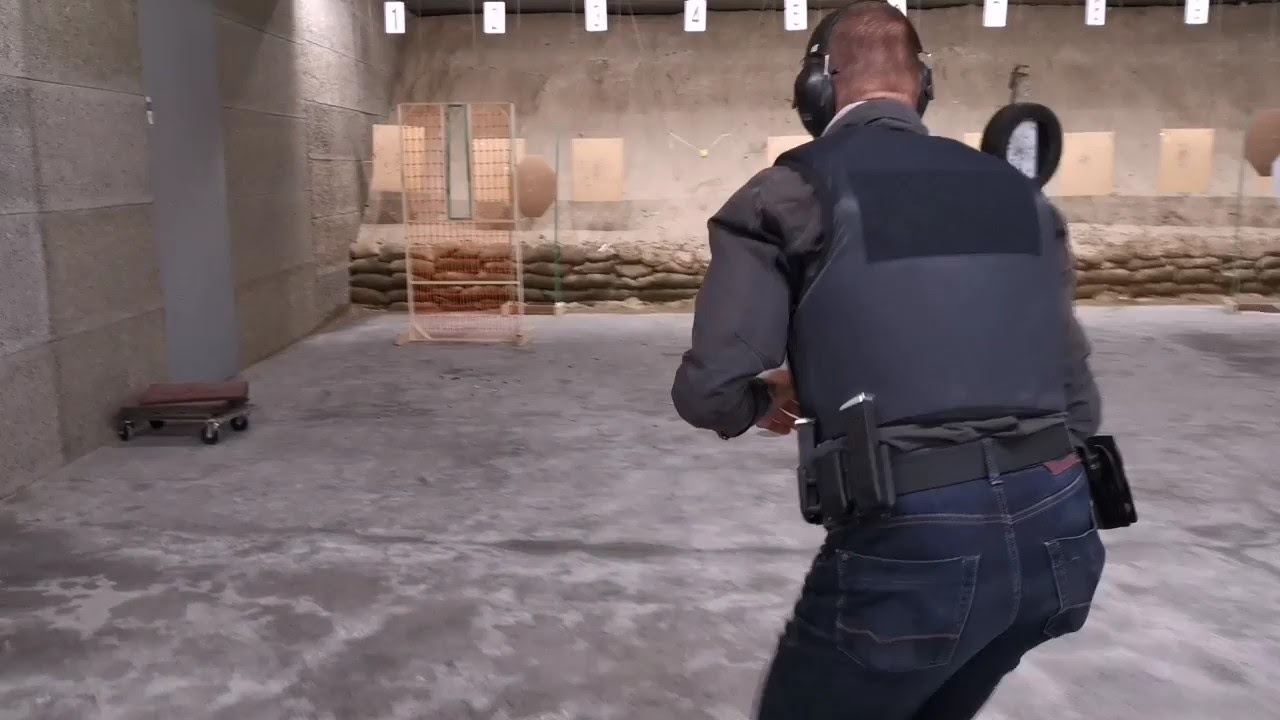In this image, we see a man standing in what appears to be an indoor gun range. He’s positioned slightly to the right of the center. The floor, made of concrete or stone, varies in color from darker shades on the bottom left to lighter shades on the right. The walls, also stone or concrete, feature large square bricks and a few openings, possibly windows. A slanted wall is visible in the background along with some well-lit areas, ensuring good visibility throughout the range.

The man, possibly a security officer, is slightly hunched forward. His right arm is mostly hidden by his side, while his left arm is reaching inward toward his chest. He’s dressed in blue jeans with a red tag on the back, a belt that could be an ammo belt, and a heavy, black, sleeveless vest, likely bulletproof, under which his shirt slightly protrudes. On his shoulder, he has a strap, and on his right belt side, there is a square object, which might be an ammo pouch or a walkie-talkie. He’s also wearing ear protection, indicating the noise level typical of gun ranges. His hair appears short, possibly shaved.

In the background, hanging targets can be seen, each marked with numbers, primarily white pieces of paper. There’s a small fence to the left with what looks like sandbags in front of it. Additional items include a potential platform made of cement bags, a cart on the left, a dolly near a silver door, and something red on the floor to the right. The target area is well illuminated, ensuring that it's easy to see and focus on the precise activities taking place.